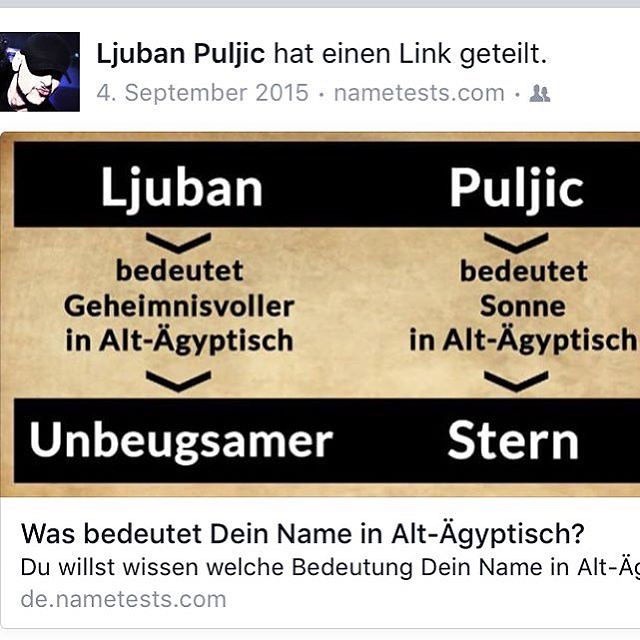The image is a digital poster, likely a social media post, primarily in German. The square image features a header at the top left with a profile picture of a man wearing a black cap, partially obscuring his eyes, and showing only his mouth and chin. To the right of the image, bold black text reads "Ljuban Puljic hat einen Link geteilt," with the date "4. September 2015" and the website "nametest.com" in light grey underneath. The top section of the square has a thick black border, while the bottom features a thin grey border.

The center section of the image is divided by black banners with white text against a tan background. On the left, a black banner says "Ljuban," followed by "Bedutet geheime Missvolle in alt-egyptisch," and an arrow pointing down. On the right, another black banner says "Puljic," followed by "Bedutet Son in alt-egyptisch," with a downward arrow, and "Stern" in white text. Below this, black text reads "Was bedeutet dein Name in alt-agyptisch?" The bottom of the image is marked by a grey text "de.nametest.com."

The layout is further accentuated with silhouettes of two people at the top near the text, providing a cohesive design indicative of a social media query or shared link related to name meanings in ancient Egyptian language.